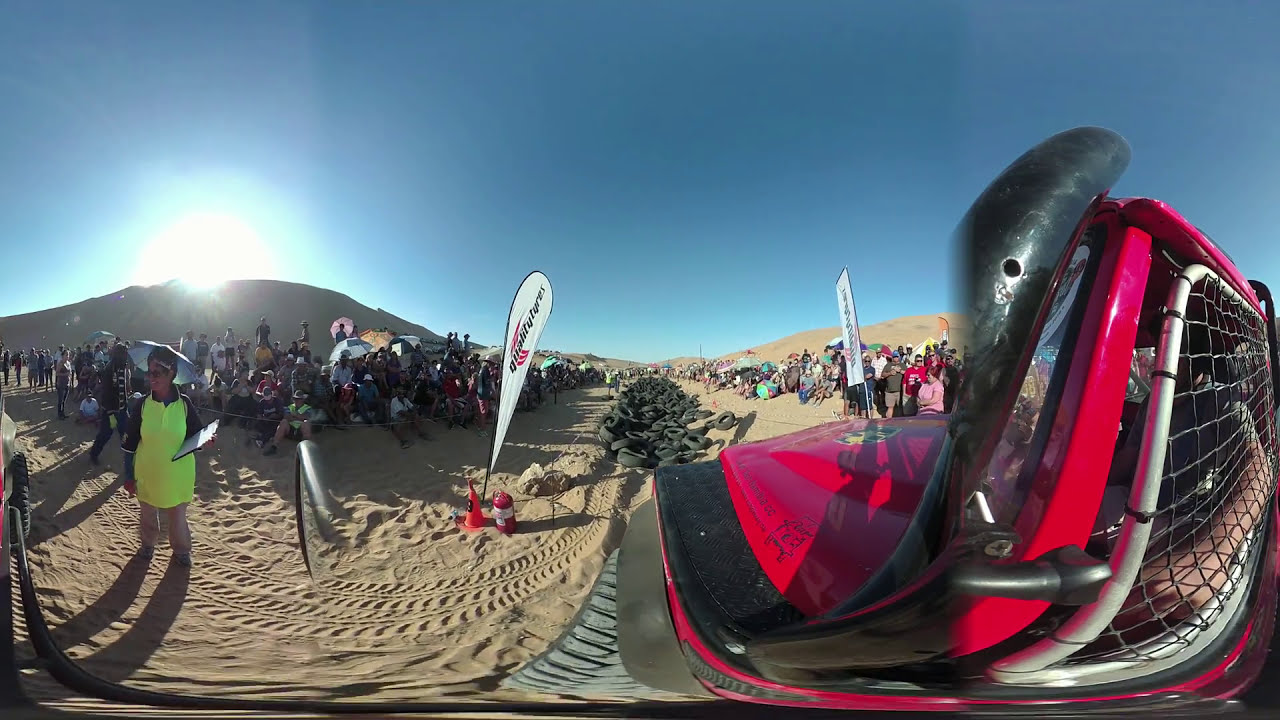The photograph captures a dynamic outdoor event set in a desert-like environment with a dramatic curved, panoramic perspective. The foreground features a partially visible red and black vehicle on the right side, somewhat distorted due to the panoramic effect. The event appears to be a motocross or off-roading competition, evidenced by the dirt track lined with tire marks and a centrally located pile of automobile tires. A conspicuous individual stands on the left, wearing a bright yellow vest, tan pants, an umbrella hat, and sunglasses, holding a clipboard. This person appears to be officiating the event. Hundreds of spectators flank either side of the track, eagerly watching the proceedings. In the background, the stark, treeless landscape rolls into small hills, with the sun either rising or setting behind one, casting a golden hue across the deep blue sky. The scene also includes scattered signs, white flags, and orange cones embedded in the sandy ground, adding further detail and depth to the panoramic shot.